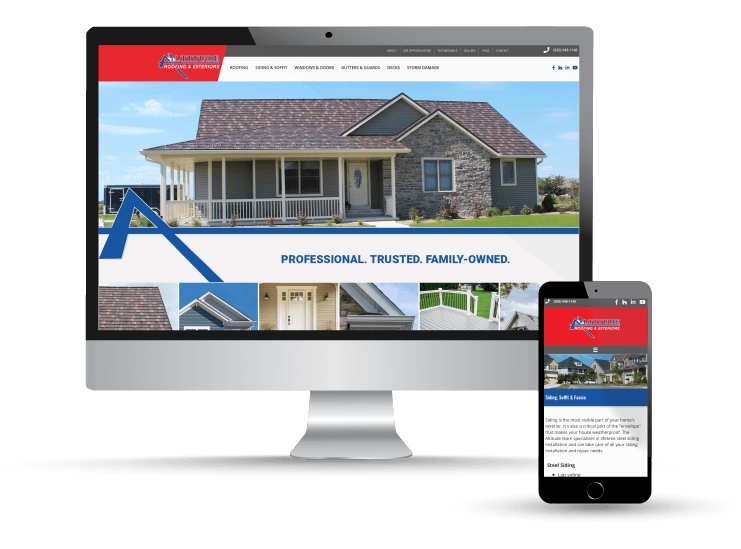This landscape-oriented card appears to be an advertisement illustrating how a website looks on both a monitor and a cell phone. In the bottom right-hand corner, there is an image of a cell phone, with its left side in black and the right side in gray. At the top of the cell phone image, there is a red section that appears to contain a business card. Directly below this, there seems to be an image related to real estate. Following this is a blue stripe, and then a white section, though the text in these sections is too small to read clearly.

In the main part of the image, positioned behind the cell phone, the upper left-hand corner features the same red logo as on the cell phone, likely related to roofing. The tabs in this section label different services such as roofing, windows, and gutters, although the text is quite small. The central focus of the main image is a detailed picture of a one-story stone house with a pointed roof made of multicolored slates in yellow, gray, and red. The house is visually appealing, with three window sections at the front, a main door, and a porch. There is a van visible on the left side behind the house, giving the scene a realistic touch. The house does not appear to have any signs indicating it's currently inhabited.